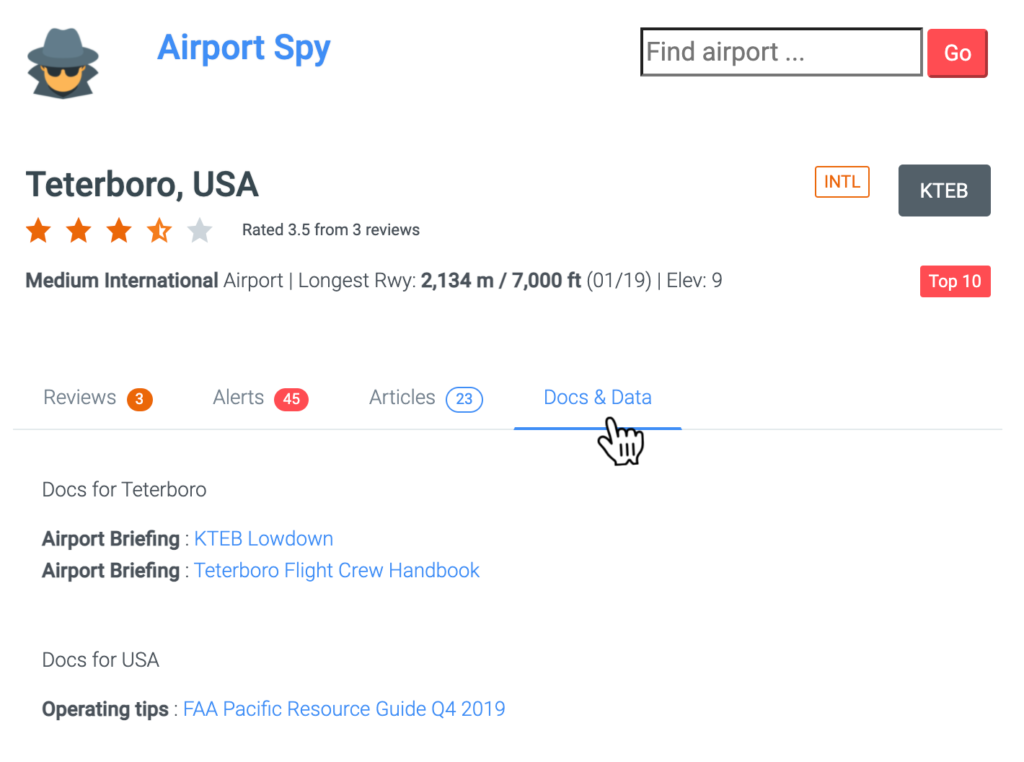The image is a screen capture of the web page "Airport Spy." At the top of the page, the title "Airport Spy" is prominently displayed. To the left of the title, there is an icon depicting a spy character, wearing a gray fedora hat, a gray coat, and black sunglasses, giving the website a covert and playful theme.

To the right of the title, a search bar is visible, allowing users to search for specific airports. The search function is accompanied by a pink "Go" button.

The main focus of the page is a search result for "Teterboro, USA." Details for this location include a star rating of 3.5 out of 5, based on three reviews. Beside the rating, there are three buttons: an orange button labeled "INTL," a gray button labeled "KTEB," and a pink icon indicating "Top Ten."

Below this information, the web page provides various pertinent details about Teterboro Airport. This includes data on the size of the runway, elevation, reviews, alerts, articles, documents, and data related to the airport. A hand icon is shown selecting "DOCS and Data," highlighting the resources available for the airport.

Additionally, there are hyperlinks for further reading, such as an airport briefing for Teterboro Airport and tips for operating at this location, providing essential information for users seeking in-depth knowledge about the airport.